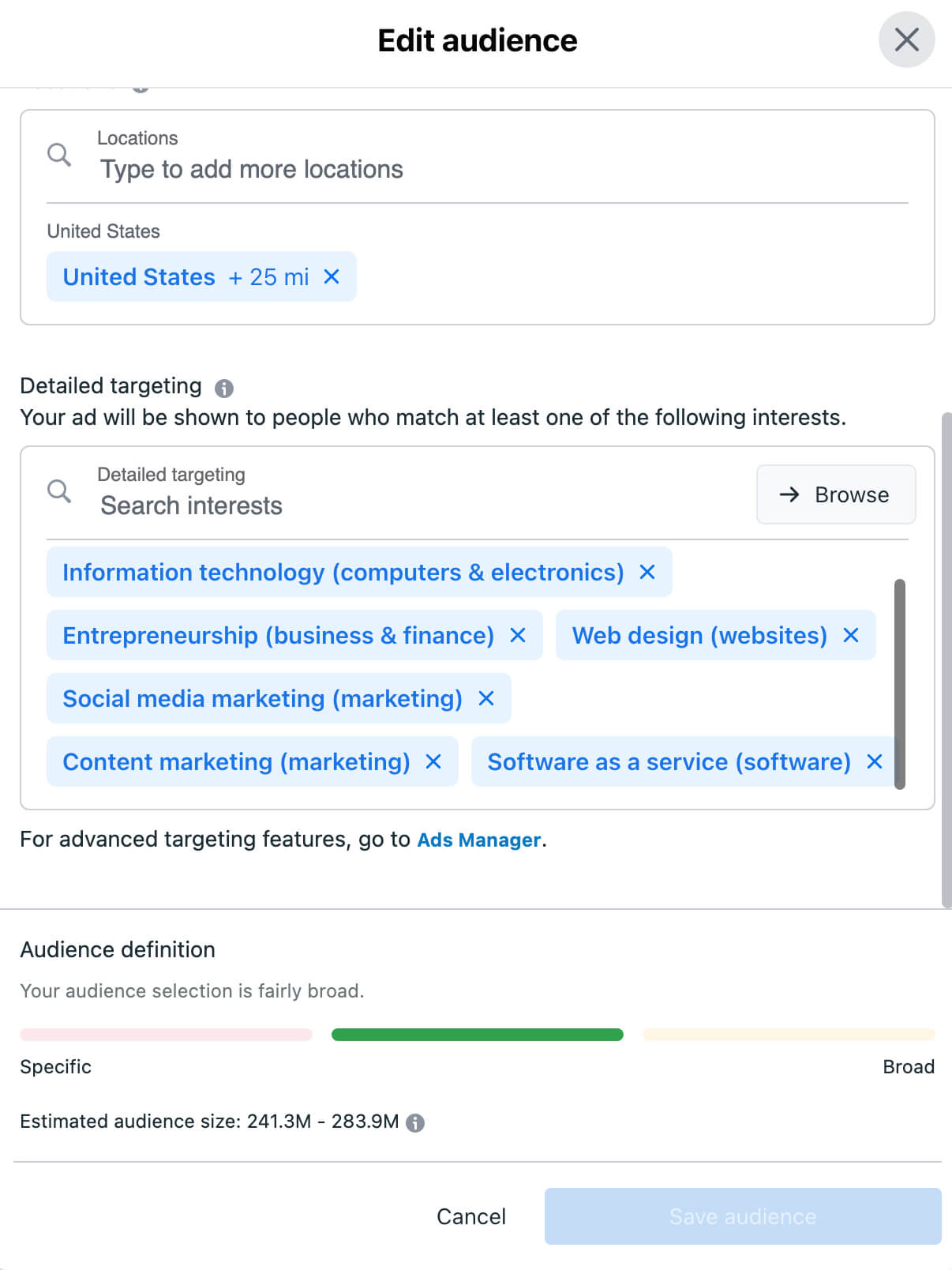The image depicts a web page interface for editing the target audience of an advertisement. At the top, the interface is labeled "Edit Audience" accompanied by a gray 'X' for closing the window.

Below this, there is a section for specifying locations, with a prompt to "Type to add more locations." "United States" is currently listed, and it's tagged with "United States + 25 miles."

In the detailed targeting section, it instructs, "Your ad will be shown to people who match at least one of the following interests." A search field labeled "Detailed targeting" allows users to search interests, with a "Browse" button (indicated by a right arrow) adjacent to it.

Several tags in blue represent the selected interests:
1. Information Technology, Computers and Electronics
2. Entrepreneurship, Business and Finance
3. Web Design, Websites
4. Social Media Marketing
5. Content Marketing
6. Software as a Service (with software in parentheses)

A note beneath this section advises, "For advanced targeting features, go to Ads Manager."

Towards the bottom, there's a section labeled "Audience Definition," which evaluates the broadness of the audience selection with a color-coded bar:
- Red indicates "Specific"
- Yellow indicates "Broad"
- Green represents the selected audience and it falls in the middle, indicating a balance between specific and broad targeting.

Finally, the estimated audience size is listed as "241.3M to 283.9M." At the very bottom, there are two buttons: a gray "Cancel" button and a blue "Save Audience" button.